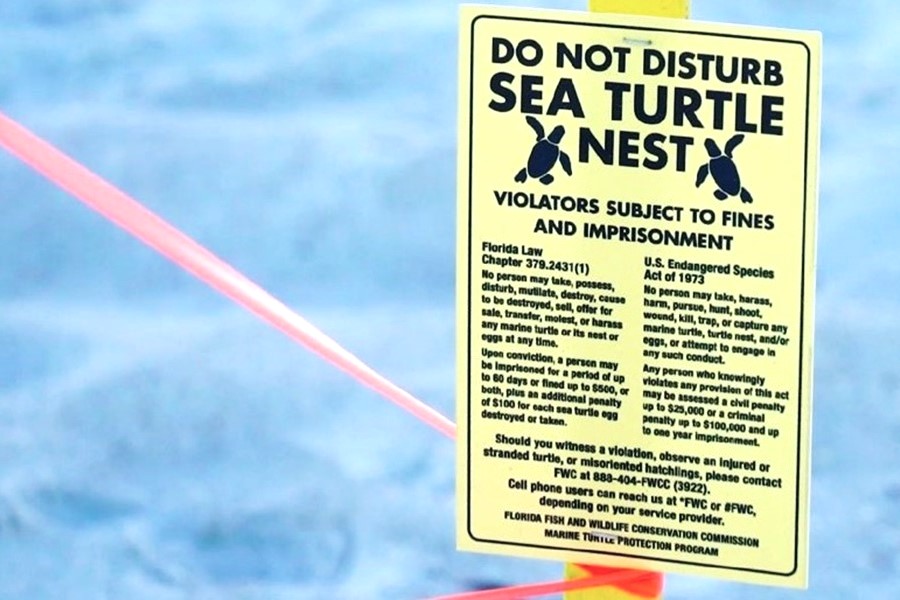The image depicts a detailed yellow sign positioned in an outdoor setting, likely near a body of water. The backdrop hints at the presence of blue water or sand, adding to the coastal environment. The sign itself is encircled by what appears to be a plastic rope or tape border. Dominating the top of the sign, in bold black text, are the words: "Do Not Disturb Sea Turtle Nest," flanked by small graphic images of black sea turtles. Directly below this, the warning "Violators Subject to Fines and Imprisonment" is prominently displayed.

The left section of the sign details Florida law Chapter 379.2431, which prohibits any form of interference with marine turtles or their nests, including actions like taking, possessing, distributing, mutilating, or selling. Offenders face penalties of up to 60 days of imprisonment, a fine of up to $500, and an additional $100 for each destroyed or taken sea turtle egg.

On the right side, the sign references the U.S. Endangered Species Act of 1973, which forbids taking, harassing, or harming marine turtles in any way, with violations resulting in civil penalties of up to $25,000 or criminal penalties reaching $100,000 and up to a year of imprisonment.

At the bottom, it provides contact information for the Florida Fish and Wildlife Conservation Commission (FWC) Marine Turtle Protection Program, encouraging the public to report any observed violations, injured or stranded turtles, or misoriented hatchlings. The provided phone numbers ensure quick and accessible reporting avenues for both landline and cell phone users. The sign is mounted on a post or cone-like structure, emphasizing its visibility and importance in the conservation efforts of sea turtles.